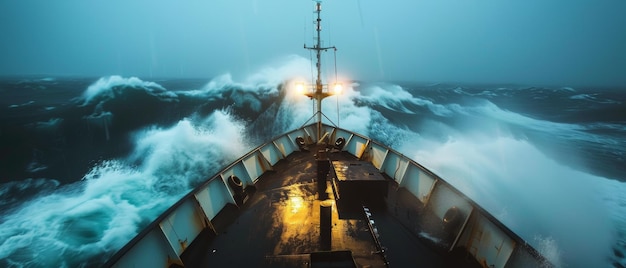This striking photograph captures the bow of an older-style commercial fishing boat battling through stormy seas. The image is taken from the captain's deck, looking forward over the ship's bow. A small mast centered at the top front of the ship is equipped with two lit floodlights, casting a reflective glow on the wet, rusty metal floor below. The boat is navigated through rough, dark gray, almost black waters, with high, choppy waves crashing against its sides, creating a misty spray around it. The ocean appears dangerously rough, with towering 40 to 50-foot waves cresting over the bow, their white caps contrasting starkly against the turbulent dark green water.

The foreboding sky above is a dark gray, shrouded in mist and rain, adding to the ominous atmosphere. The photograph highlights the bow's essential details, showing rubber tires folded inward, used as bumpers, and several life preservers along the white-rimmed edges. A box sits to the right of the mast, likely containing anchor chains or related materials, hinting at the boat's utilitarian purpose. Despite its slightly rusted appearance, the ship pushes forward resiliently through the storm, a testament to the harsh realities of life at sea.